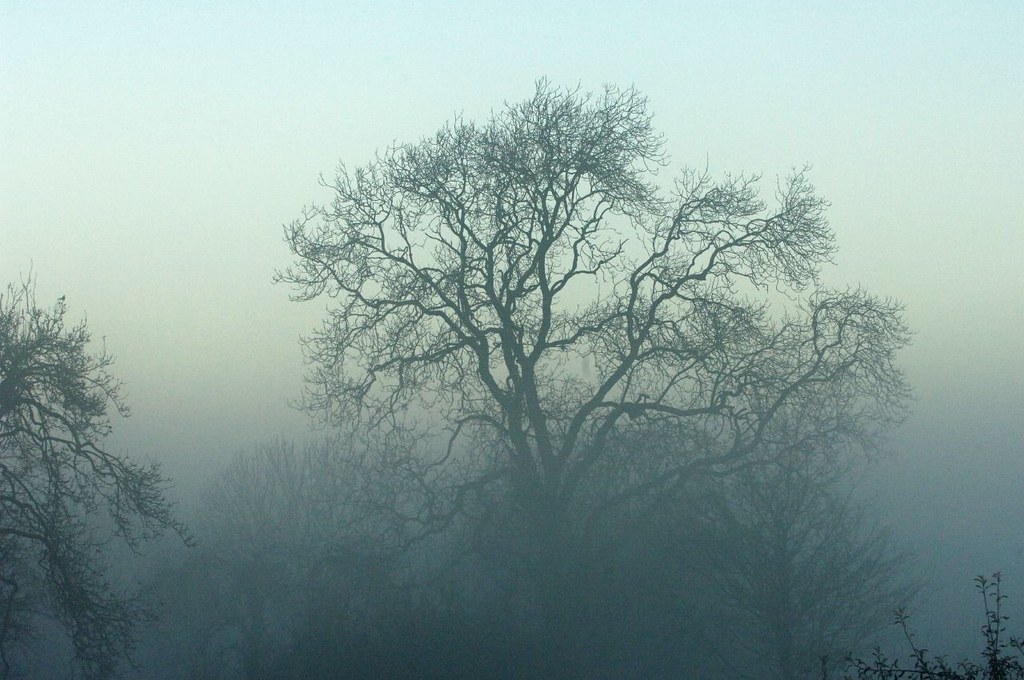This image captures a striking, fog-laden outdoor scene centered around a large, leafless tree with expansive, intricate branches that meander upward through the fog. The sky transitions from light blue at the top to a near-white cloud deck closer to the horizon, adding to the overall ethereal atmosphere. The fog partially obscures the tree, rendering it a dark gray silhouette against the hazy backdrop. In the bottom right corner, there are dark, scratchy plants, providing additional texture to the image. Surrounding the central tree are other trees and branches, some with leaves, but they are faintly visible through the pervasive fog, enhancing the scene's mysterious and layered quality. The colors present in the photograph include shades of white, blue, gray, and black, contributing to the serene yet somber mood.